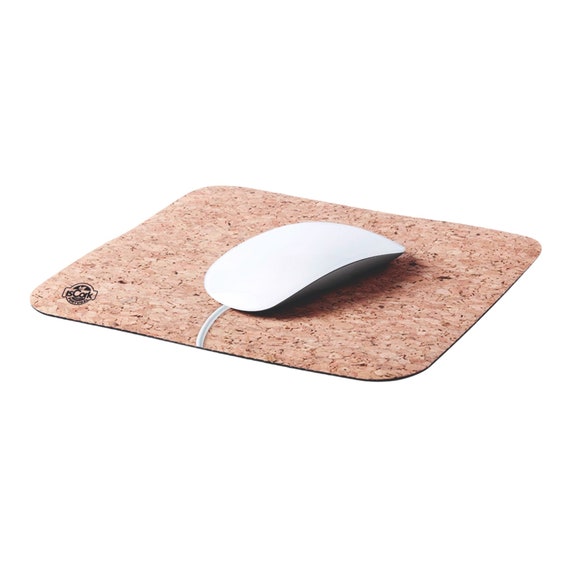The image features a professional photo of a white computer mouse with a gray underside, positioned on a brown corkboard-like mouse pad. The mouse pad has the texture and appearance of cork, similar to a corkboard wall used for pushpins. The mouse is centered on the pad and has a visible cord trailing off, although part of it is cut off at the edge of the mouse pad. A small, black round logo with the word "cork" is located in the bottom left corner of the mouse pad. The entire scene is set against a white background, giving the object a floating appearance. The overall color scheme includes white, black, gray, and various shades of brown. There are no other elements, such as text or living beings, in the image.